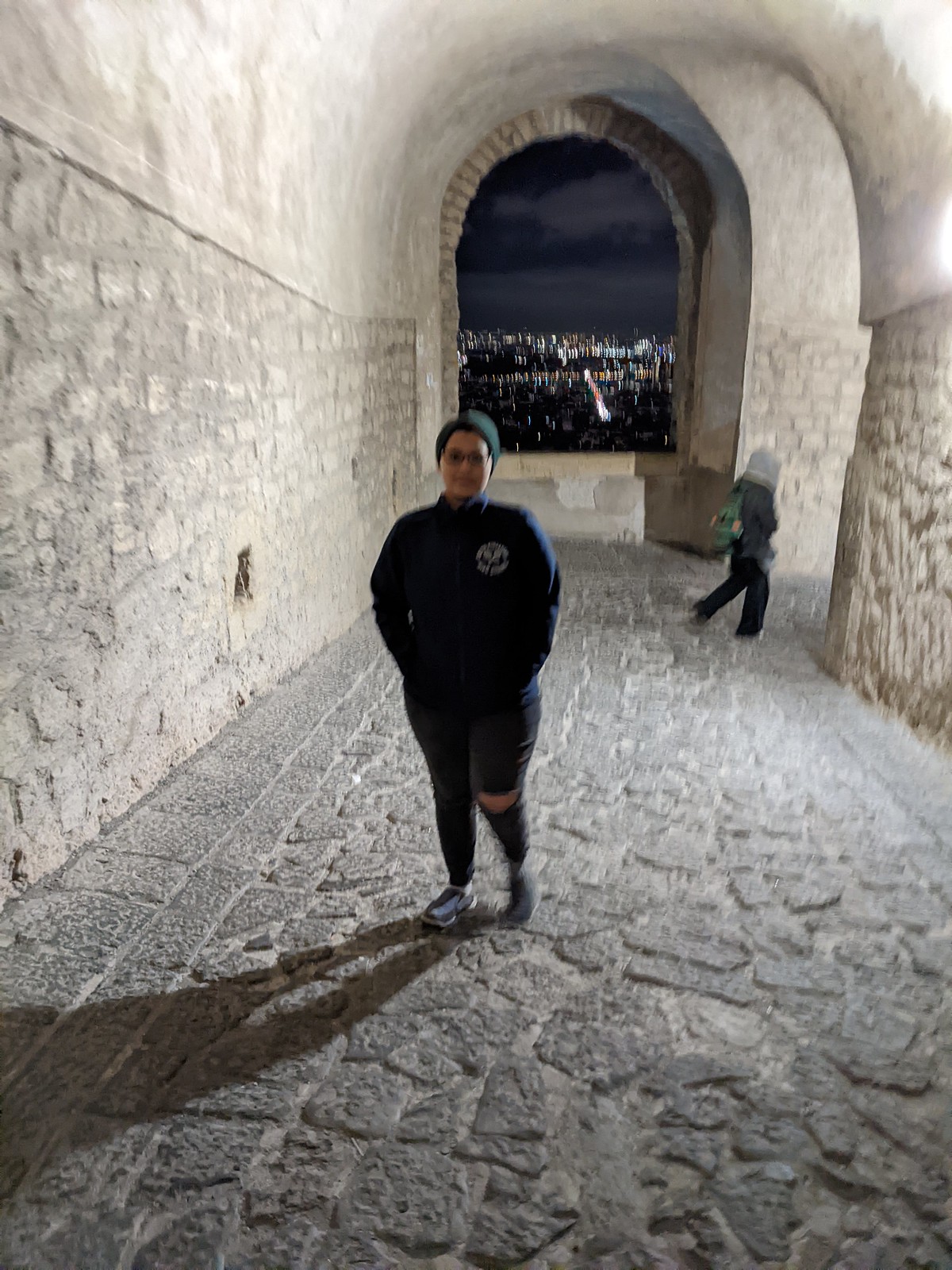Captured during the night, this image showcases the interior of a well-lit, tunnel-like structure within an old building. The architecture, characterized by a series of plastered arches and cobblestone paths, leads the eye towards an open arched window that reveals a distant cityscape sprinkled with lights beneath a dark, cloudy sky.

Central to the photograph stands a female figure dressed appropriately for chilly weather. She wears a jacket and a stocking hat, paired with long pants that feature a fashionably ripped design at the left knee. Her hands rest casually in her pockets. To the right, another figure dressed in a gray top and a white hooded scarf walks away, carrying a blue backpack and sporting dark pants.

The aged walls of the structure, composed of cemented white and gray stone, alongside the meticulous detailing of the repetitive arches, contribute to the historic and almost ethereal ambiance of the scene, creating a vivid contrast to the modern cityscape visible in the background.